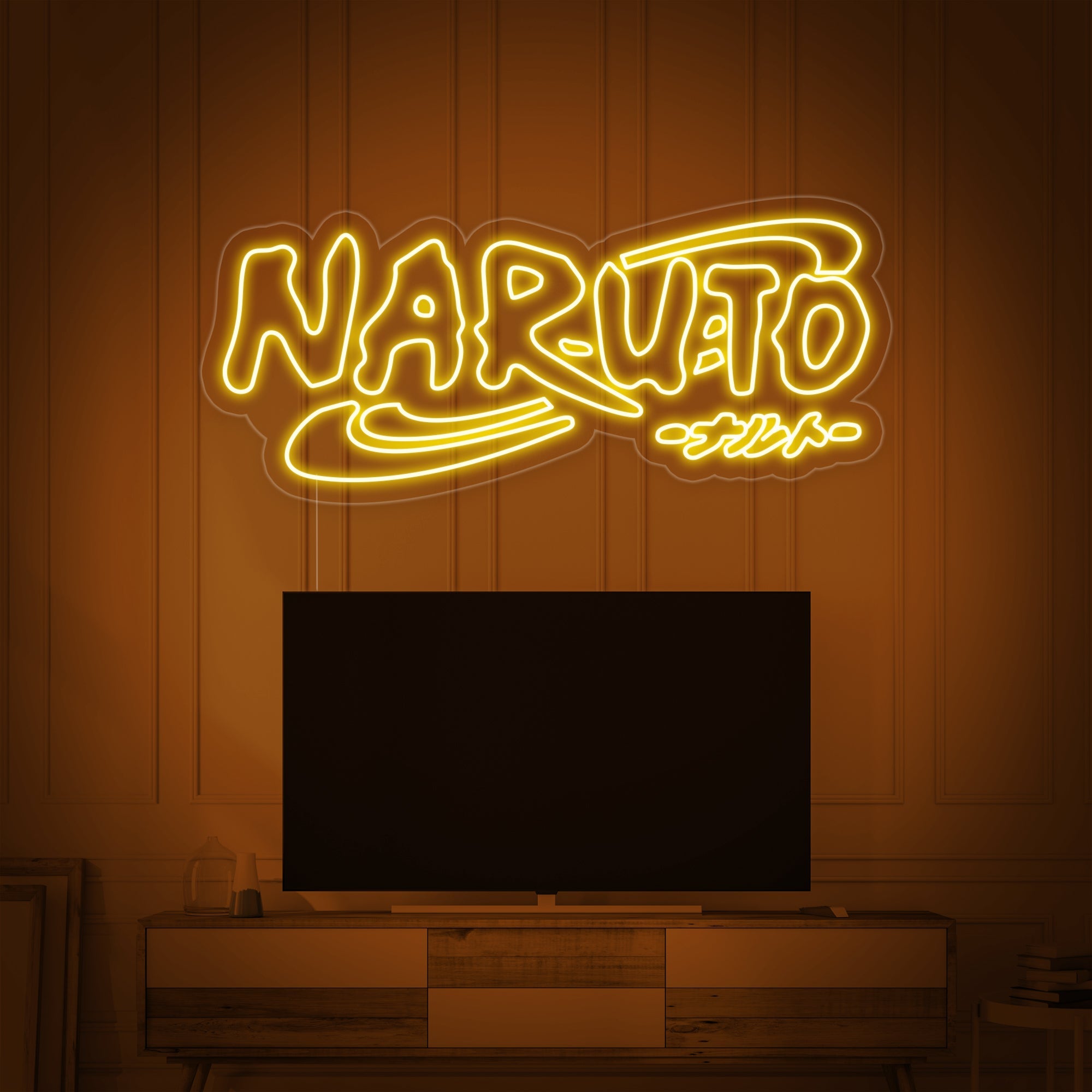The image depicts an interior wall clad with evenly spaced light brown wood panels. Mounted on this wall is a flat-screen TV with a black screen, sitting atop a wooden stand resembling a dresser. The front of this stand is decorated with alternating light and dark brown wooden panels arranged in a checkerboard pattern. Above the TV, a bright yellow neon sign glows with the word "Naruto" written in a wobbly font, accompanied by additional text in what appears to be another language, likely Chinese, below it. The bottom left corner of the image hints at a partial photo or object leaning against the wall, while the bottom right features an end table holding four or five books. The composition of the scene is completed by two yellow curvy check mark lines flanking the neon sign. The overall color palette includes brown, black, and yellow.